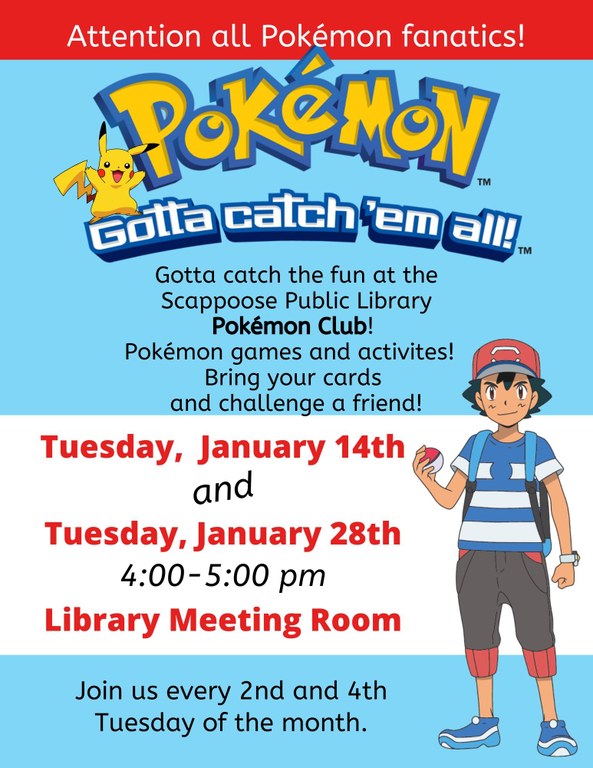The image showcases a vibrant, well-designed advertisement for a Pokémon-themed event at the Skippo's Public Library. 

The top of the ad features a bold red bar with white text that reads, "Attention all Pokémon Fanatics!" The iconic Pokémon logo, rendered in its classic blue and yellow color scheme, is prominently displayed below this header. Standing next to the logo is Pikachu, the beloved mascot of the franchise. Below the logo, the famous tagline "Gotta Catch 'Em All!" is imprinted in energetic blue lettering.

Directly beneath this, the main body of the ad contains details about the event: "Gotta catch the fun at the Skippo's Public Library Pokémon Club!" It further outlines activities such as Pokémon games and challenges. Attendees are encouraged to bring their cards and challenge friends. The event dates and times are specified as Tuesday, January 14th, and Tuesday, January 28th, from 4:00 PM to 5:00 PM, taking place in the library's meeting room. It also mentions that the club meets every second and fourth Tuesday of the month.

To the right of the text, there is a colorful depiction of Ash Ketchum, a central character in the Pokémon series, adding a touch of dynamic energy to the flyer. 

The ad maintains a cohesive color scheme of blue, white, and red throughout, with the red top bar providing a striking contrast to the blue and white sections containing the text.

Overall, the advertisement appears very well-crafted and inviting, promising an exciting and engaging experience for children and Pokémon enthusiasts alike.